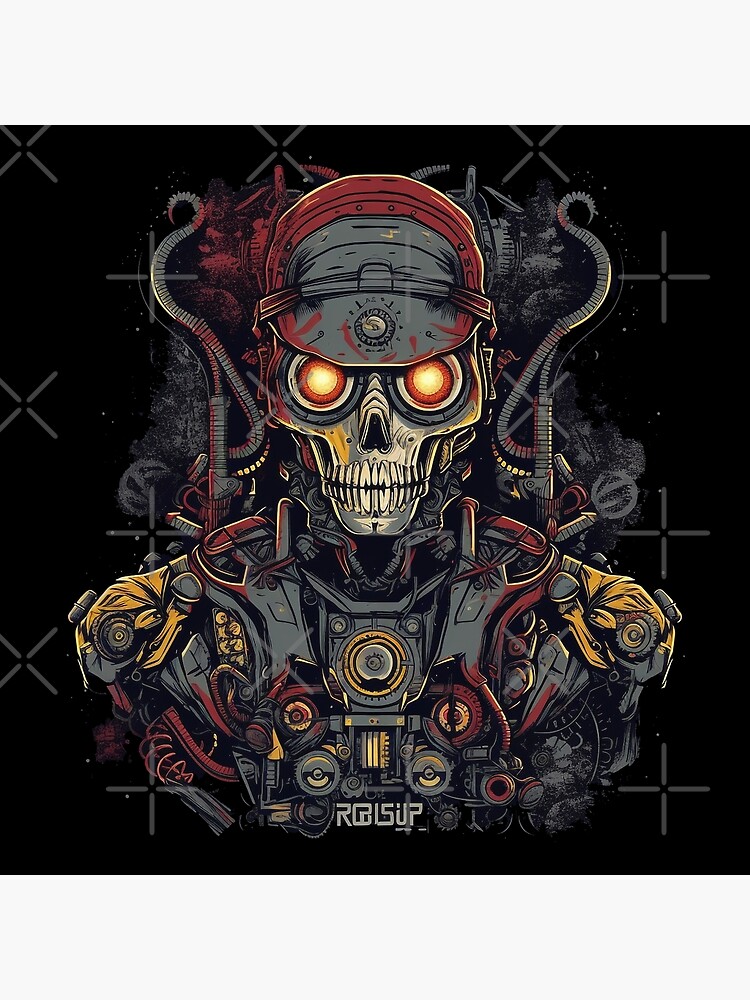The artwork is an intricate, edgy cartoon drawing of a demonic skeleton-like robot soldier. The skeleton's head features metal components, including a metallic nose, teeth, and orange-red glowing, goggle-like eyes. It wears a hat that is a mix of gray and red. The visible part of the body – the shoulders and chest – appears to be made of a complex arrangement of mechanical parts, including gears, valves, and hoses that connect the shoulders to the head area. The primary colors in the image are red, orange, yellow, gray, and white, giving it a dark and menacing vibe. The background is black with gray X's and crosses scattered throughout, adding to the overall ominous atmosphere. The artist’s name, "RBI sup," seems to be subtly integrated into the background design, though it’s challenging to discern clearly due to the stylized nature of the image.